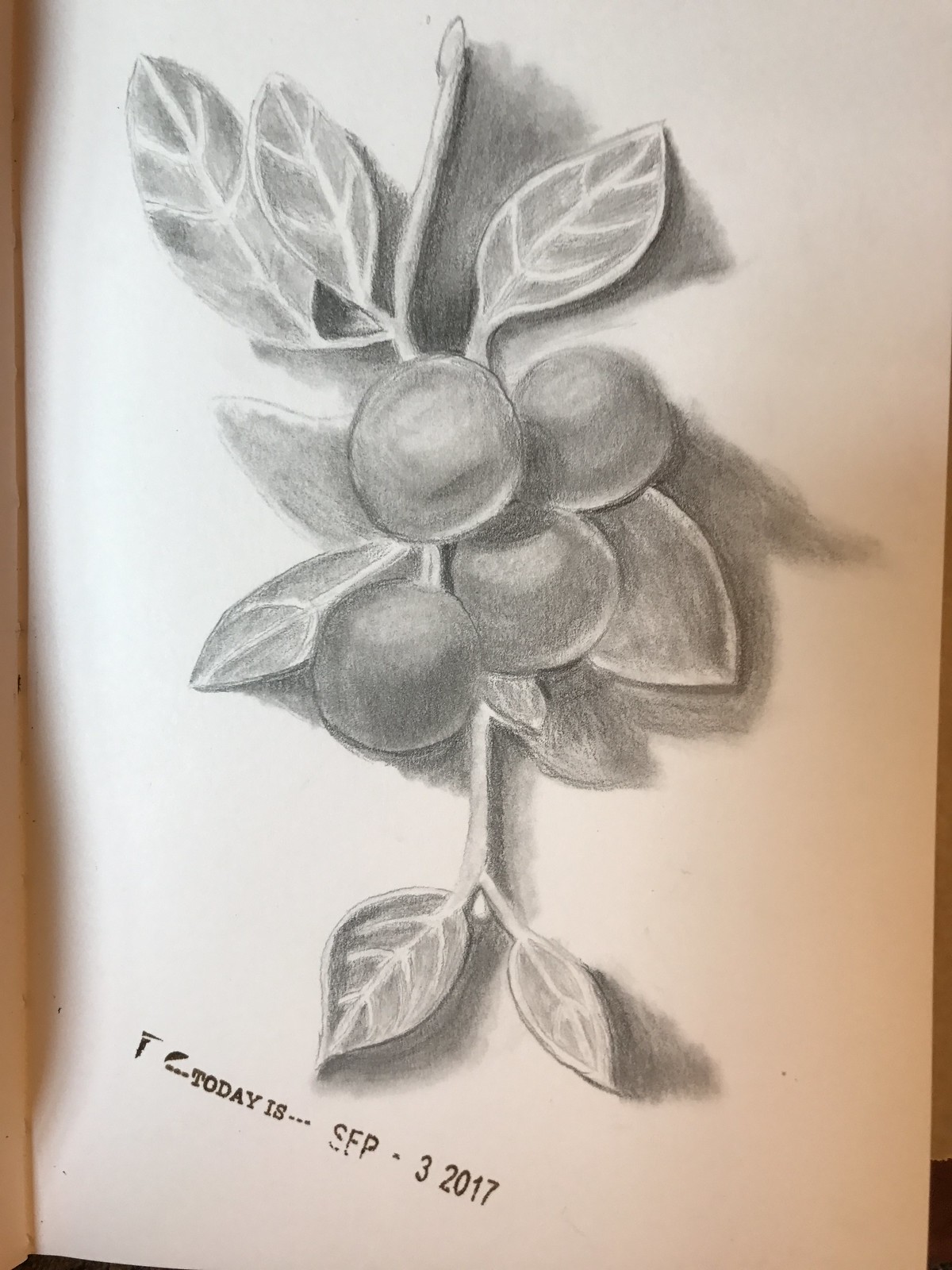This image showcases a detailed pencil drawing on white sketchbook paper, likely an indoor photograph of the open book. The central subject is a plant with a complex network of vines and branches. The plant features multiple vines with numerous leaves sprouting from them. The main vine in the center extends both upwards and downwards, with the top part tapering into a small point and the bottom part splitting into two branches that carry leaves.

At the heart of the vine structure are four round fruits, shaded intricately on the bottoms, suggesting a light source from the left side. These fruits may resemble cherries, apples, or similar small fruits, each depicted with a naturalistic shading that conveys depth and form. Two of the fruits are positioned to the left of the center, and two on the right, adding a balanced symmetry to the composition. The left side possibly involved light pastel or apricot tones over the paper, adding a subtle hue to the monochrome drawing.

Towards the bottom of this artistic piece, a date stamp is visible. It reads in bold capital letters, "Today is September 3rd, 2017," slightly slanted from the upper left to lower right of the image. The entire drawing is well-executed, with detailed shading and shadow effects, giving a three-dimensional feel to the leaves and fruits. There are no other texts or print on the image, focusing the viewer’s attention entirely on the botanical subject.